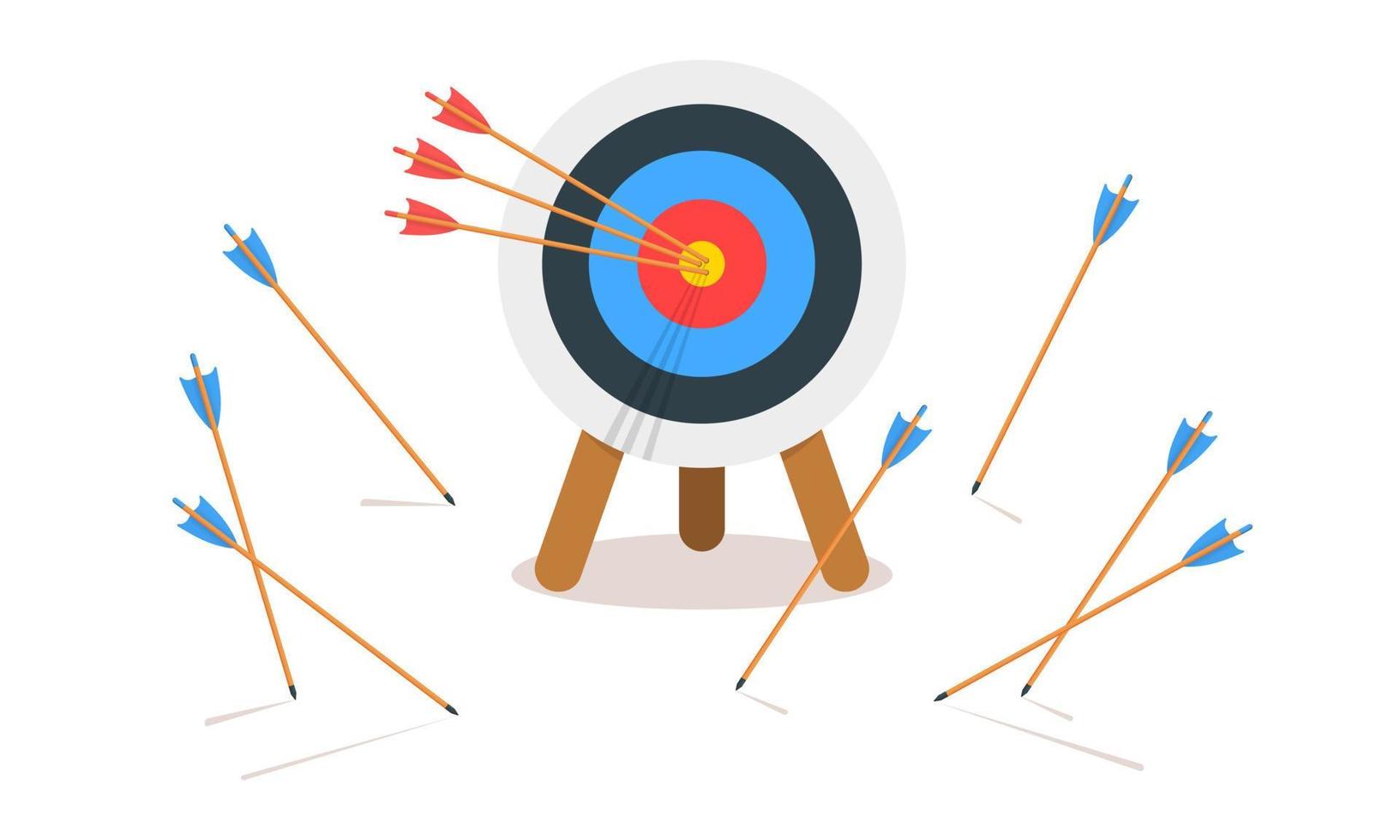The image features a stylized graphic artwork of a circular bullseye target mounted on a brown wooden tripod stand. The target comprises several concentric rings: a white outermost ring, followed by a black ring, a dark blue ring, a royal blue ring, a red ring, and a yellow center. Three red-tipped arrows are embedded in the yellow bullseye, casting shadows on the target. Scattered around the target on a white background are seven arrows with blue tips: three lie to the left on the ground, and four are on the right, with two of them crossing each other. The target and the arrows cast slight shadows, adding depth and dimension to the image.